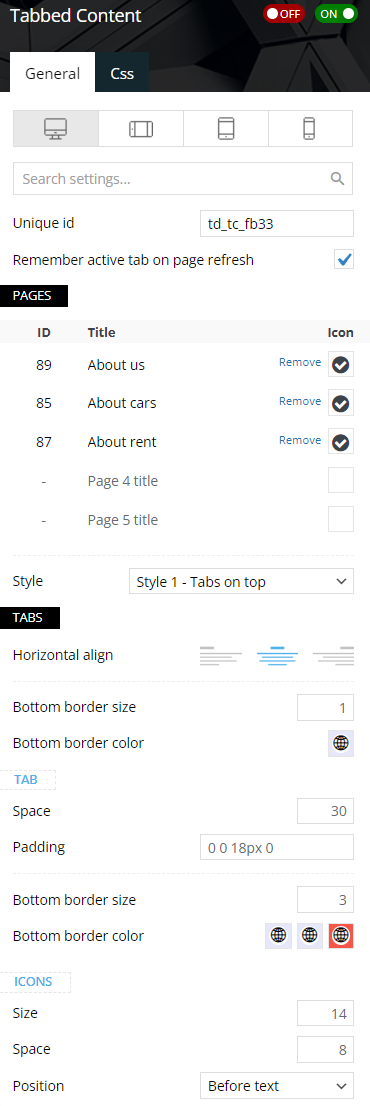This image is a screenshot from a phone displaying a detailed interface, primarily featuring a CSS editor. The top inch of the screen has a black background with the words "tapped content" in bold white font on the top left corner. Extending from the left, there is a green tab with the word "on" in white, positioned to the right of a white circle. Adjacent to it on the left is a red tab with a white circle on the left side and the word "off" in white.

Below these tabs, a small white rectangle protrudes into the black border. The word "general" in black letters is visible just inside the white rectangle. Moving back into the black border, the word "CSS" is written in white, indicating the section of the editor in use. There are four clickable tabs below this title: the first tab is gray, and the next three are white. The icons on these tabs represent a laptop, a tablet, and two cell phones, respectively. Beneath these tabs is a search bar labeled "unique ID."

To the right, there is a rectangle containing a specific unique ID. Below this, the phrase "remember active tab on page refresh" is written in black, with a blue-checked square to its right. The whole page has a white background, contrasting with sections of black where additional information is presented.

Further down, there is a black tab labeled "pages," under which numbers representing IDs and corresponding titles are listed. To the right are squares, with the first three checked and labeled "remove" in blue. The bottom two squares are empty.

On the left side, a section labeled "style" and another drop-down menu also labeled "style" are noted. Below this, a black tab titled "Tab" lists ten clickable options; "Tab" and "icons" are in blue, while the rest are in black. On the right side are rectangles and squares with numerical data, providing additional functionality and information.